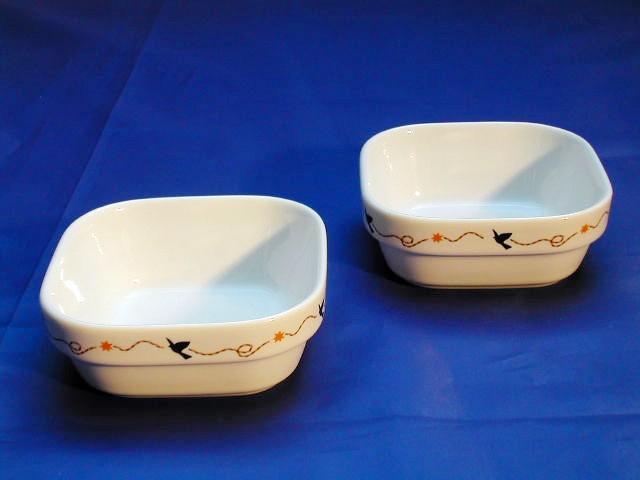The image depicts two small, white ceramic cups, nearly squarish or rectangular in shape, each adorned with an intricate design around the outer rim. The design features a bird, resembling a dove, accompanied by a twisting, orange-reddish string that forms a star shape and then continues. This pattern – bird, string, star, string – repeats both in front and behind the bird. These cups sit atop a royal blue cloth that shows signs of creasing on the left side, casting shadows due to the lighting. Together, the elements in the image suggest a balance of simplicity and detailed craftsmanship.